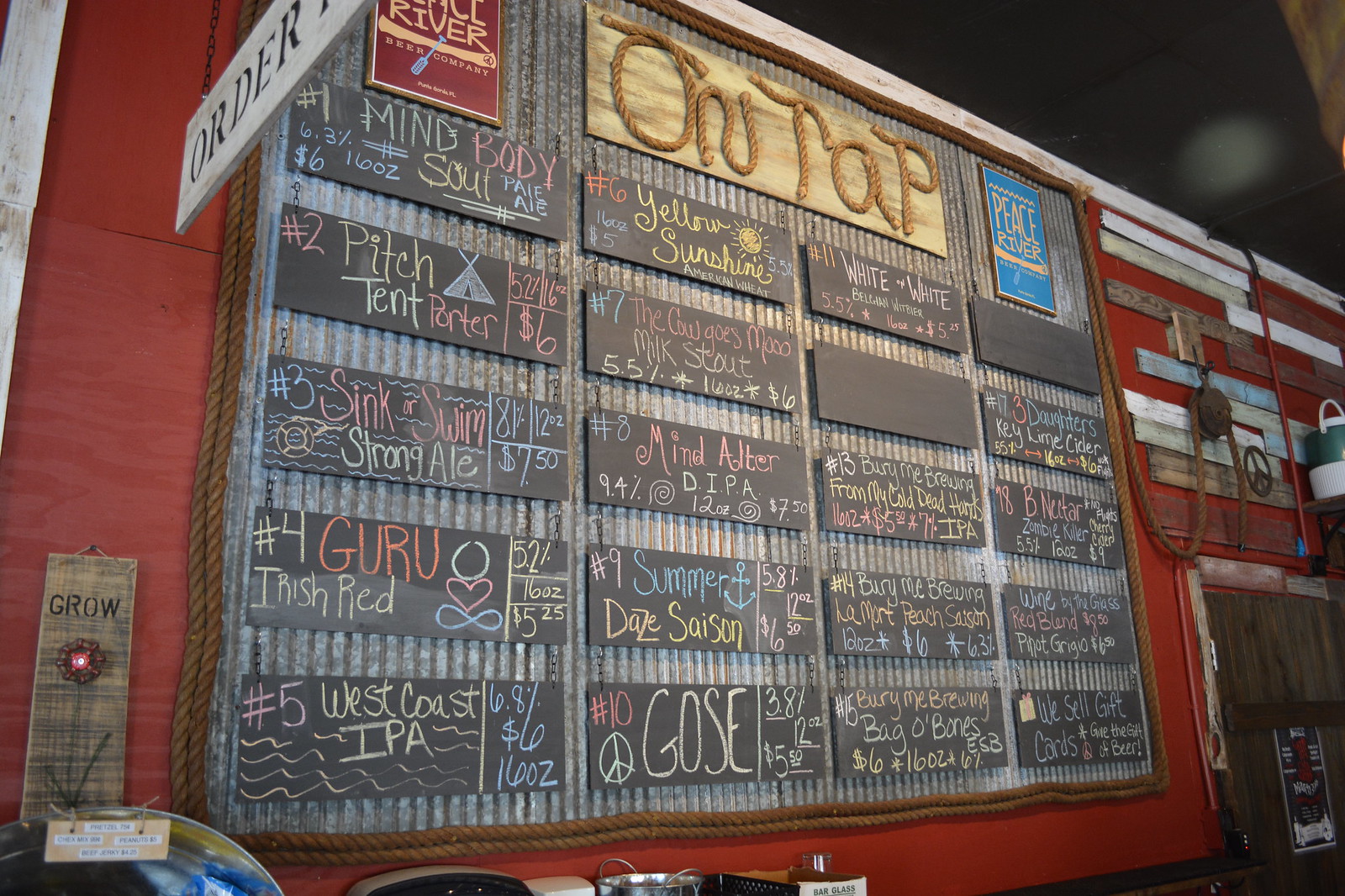This indoor photograph captures a rustic, nautically-themed brewery with a striking red wall. Mounted on the wall are 20 small chalkboards, each detailed with the various beers available on tap, written in vibrant chalk colors like blue, red, yellow, and green. The top of the display features a wood sign with "On Tap" spelled out in rope, flanked by the name "Peace River Beer Company." Each chalkboard lists a numbered beer, including options such as "Mind, Body, Soul Pale Ale" (#1), "Pitch Tent Porter" (#2), "Sink or Swim Strong Ale" (#3), "Guru Irish Red" (#4), and "West Coast IPA" (#5). Additional noted selections include wheat beers, milk stouts, and saisons. An "Order" sign hangs from chains, indicating where to place your drink selection. This inviting setup emphasizes a variety of brews in a coastal, artisanal ambiance.